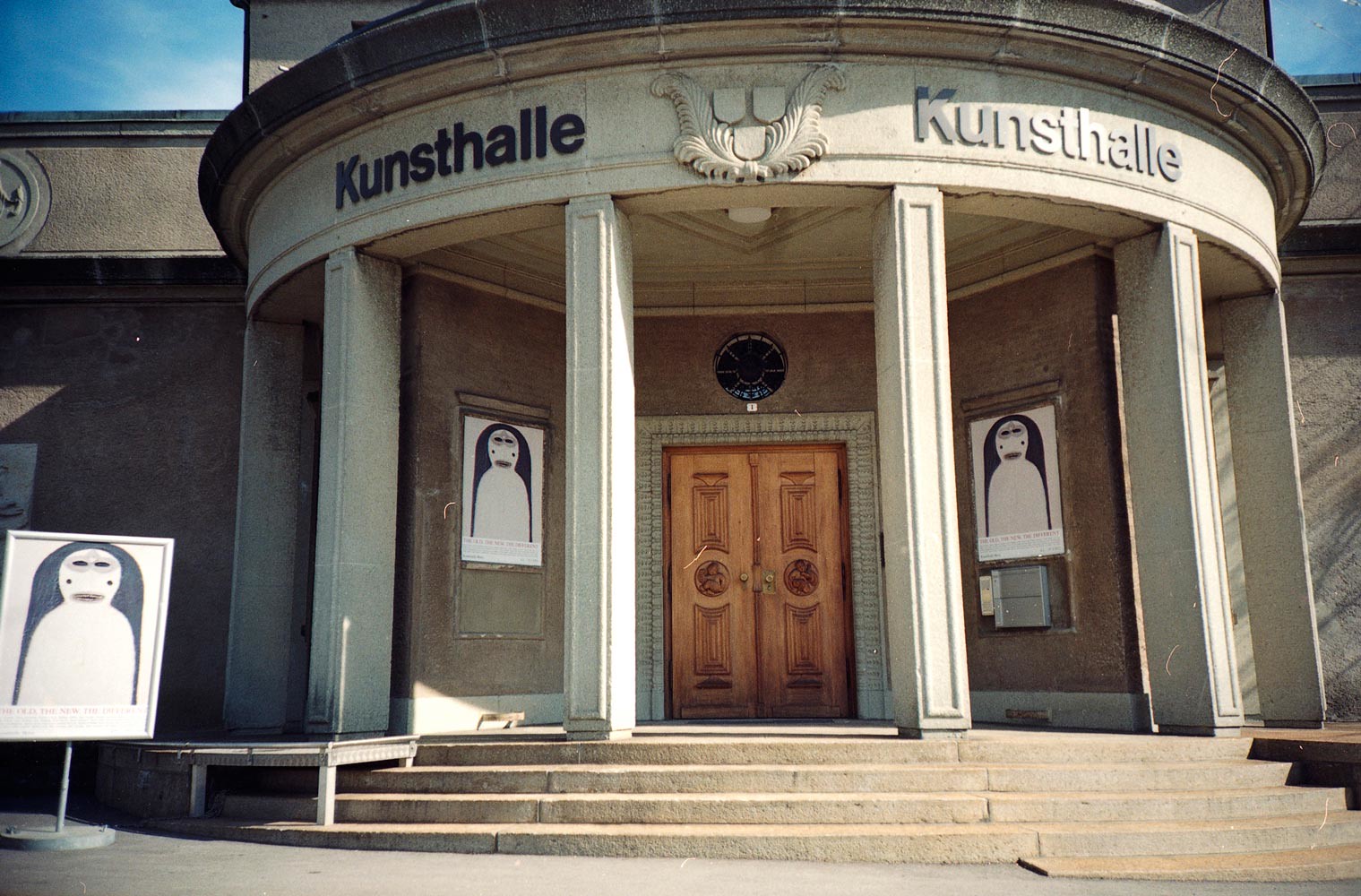The image depicts an outdoor scene featuring a building with ancient architectural elements, predominantly grey in color. The central focus is on a set of large, closed double wooden doors, brown in color, which are accessible via a series of stairs leading up from a circular patio. Flanking these doors are imposing columns that add to the grandeur of the entrance. Above the doors, there is an emblem or crest, which seems to display three shields with feathers on either side. Surrounding this crest, the letters "Kunststahl" or "Kunz Hall" are prominently displayed.

The walls of the building are adorned with posters showing an alien-like cartoon character, white in color with black eyes and a grey mouth. These posters are strategically placed, with two on either side of the doorway and another to the left of the building. The clarity of the image is high, with all elements distinctly visible.

The overall visual setting is bright, suggesting a daytime capture with plenty of natural light and a clear blue sky overhead. The mix of detailed stonework, historical architectural design, and contemporary cartoon posters presents a visually intriguing contrast. The scene is devoid of people, emphasizing the building's stark and stately presence.